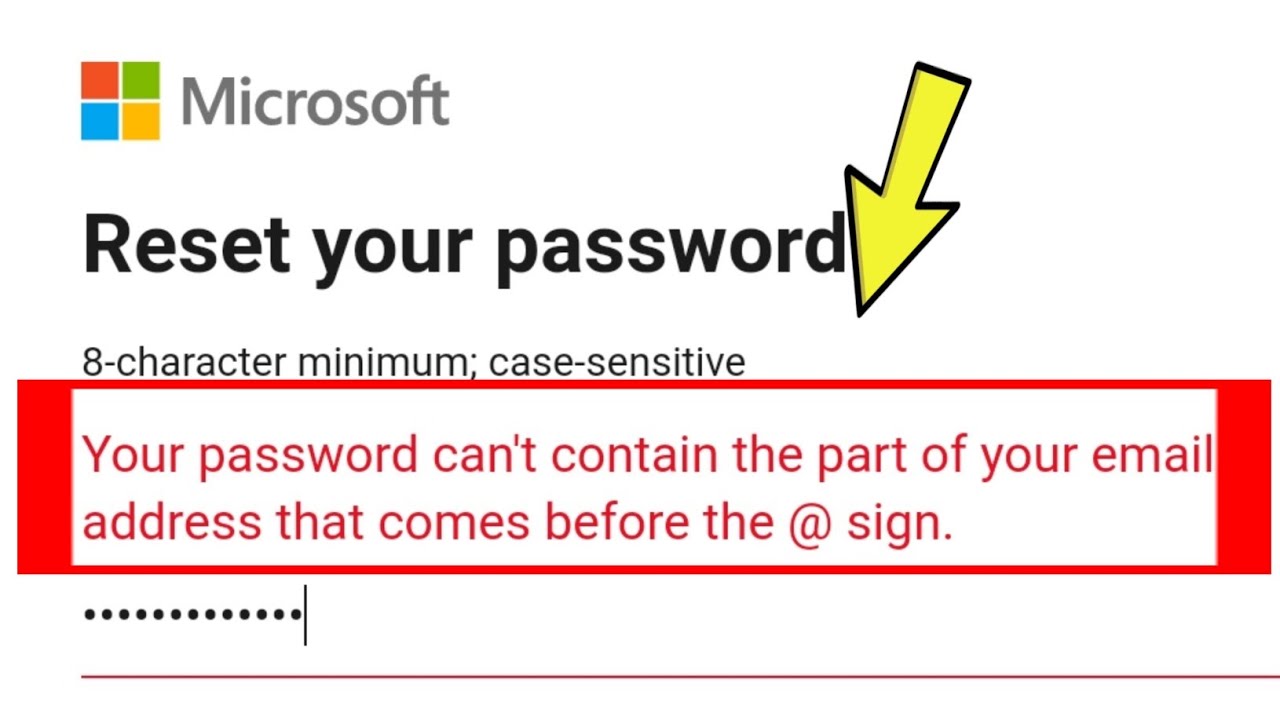Screenshot of a Microsoft password reset screen on a white background. The prominent Microsoft logo, with its emblematic red, green, blue, and yellow squares, appears at the top. Below the logo, the heading "Reset your password" is displayed in bold black text. A yellow arrow highlights an error message contained within a red rectangle. The error message reads, in red text, "Your password can't contain the part of your email address that comes before the @". Above this error, a set of password requirements is outlined in black text: "8 character minimum, case sensitive". Below these instructions, thirteen dots represent the entered password, with a cursor flashing at the end of the dots. A red underline appears at the bottom of the screen, indicating an input field or error state.